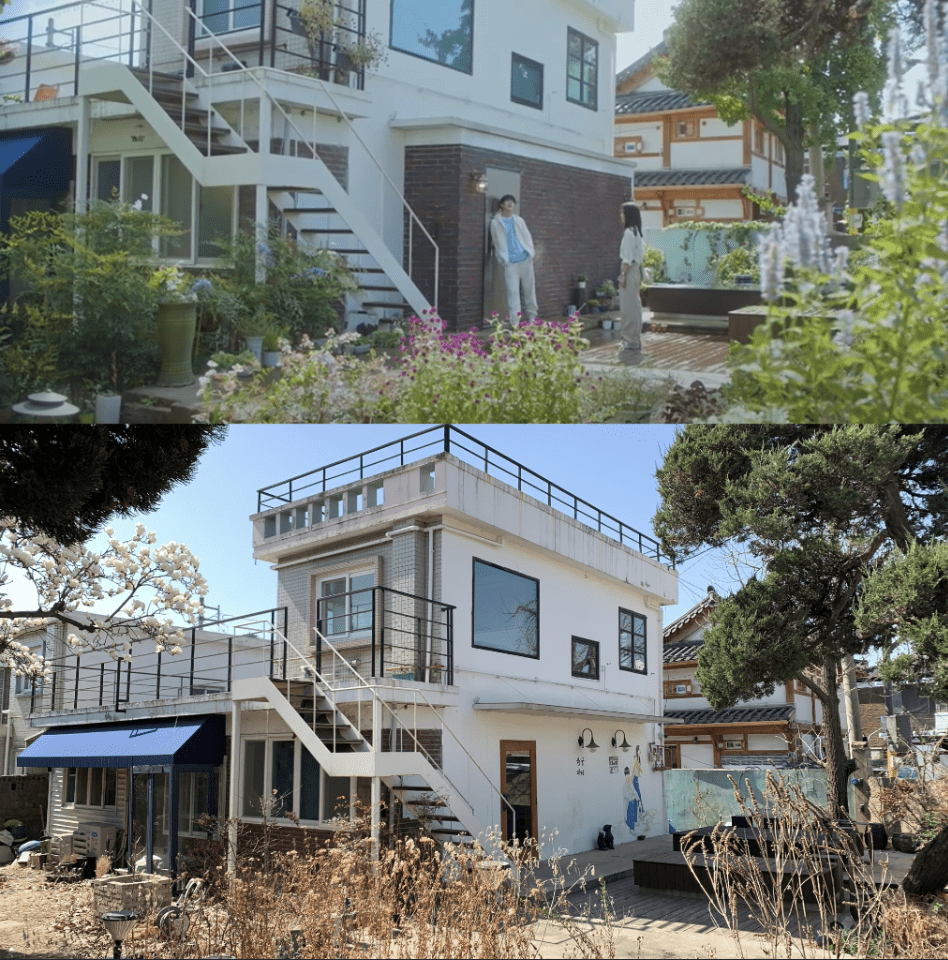The square image presents two photographs of a distinctive white two-story house. In the top image, two individuals stand beside a brick wall next to a door. The man, wearing a white jacket, white pants, and a blue t-shirt, leans casually against the house. The woman, dressed in khaki pants and a white top, gazes at him, with her dark shoulder-length hair and left wrist watch visible. This scene is set in a lush environment with various plants, suggesting a warm climate. A set of stairs leads up to a deck at the back of the house, and a green tree extends from the right side of the image. An additional house and traditional-style buildings are visible in the background.

The bottom photograph, which occupies a larger portion of the frame, shows a similar angle of the house, but without the people or the brick wall. Instead, a glass door and two wall-mounted lights are prominent features. The environment appears drier, with dead grass and patches of dirt, indicating a change of season. The house’s structure includes large upper windows with black framing and a railing on the top level, suggesting access to a rooftop area. Both images provide a comprehensive view of the house's architecture and seasonal differences in the surroundings.